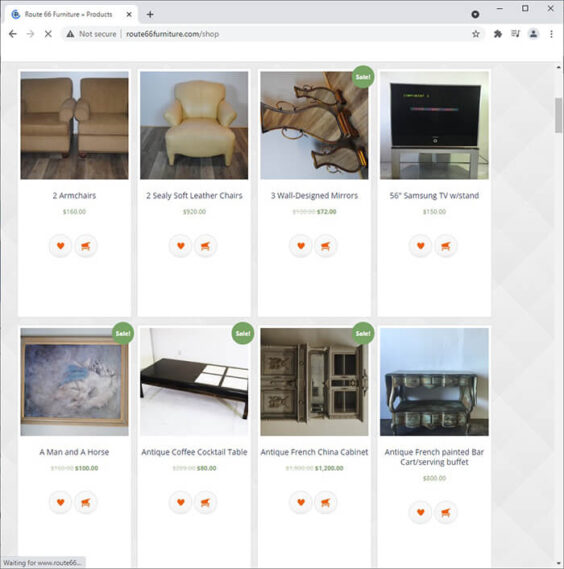The image displays a webpage from a site entitled "Route 66 Furniture and Products," as seen from the open browser tab in the upper left-hand corner. The webpage’s URL reads "route66furniture.com/shop," with a notice indicating the site is "Not Secure" in the browser's address bar. There are navigation arrows and a close button beside the URL.

The main section of the image showcases a collection of furniture items arranged in two rows, each featuring four pieces.

Top row, from left to right:
1. A pair of beige armchairs.
2. A single tan armchair.
3. Decorative wall mirrors, marked with a green "Sale" circle.
4. A 56-inch Samsung TV mounted on a stand.

Bottom row, from left to right:
1. A painting depicting a man and a horse.
2. A low black antique coffee table.
3. An antique French china cabinet.
4. An antique French painted bar cart serving buffet.

This website specializes in high-end, rare, and one-of-a-kind items, as indicated by the uniqueness and apparent value of the antique pieces displayed.